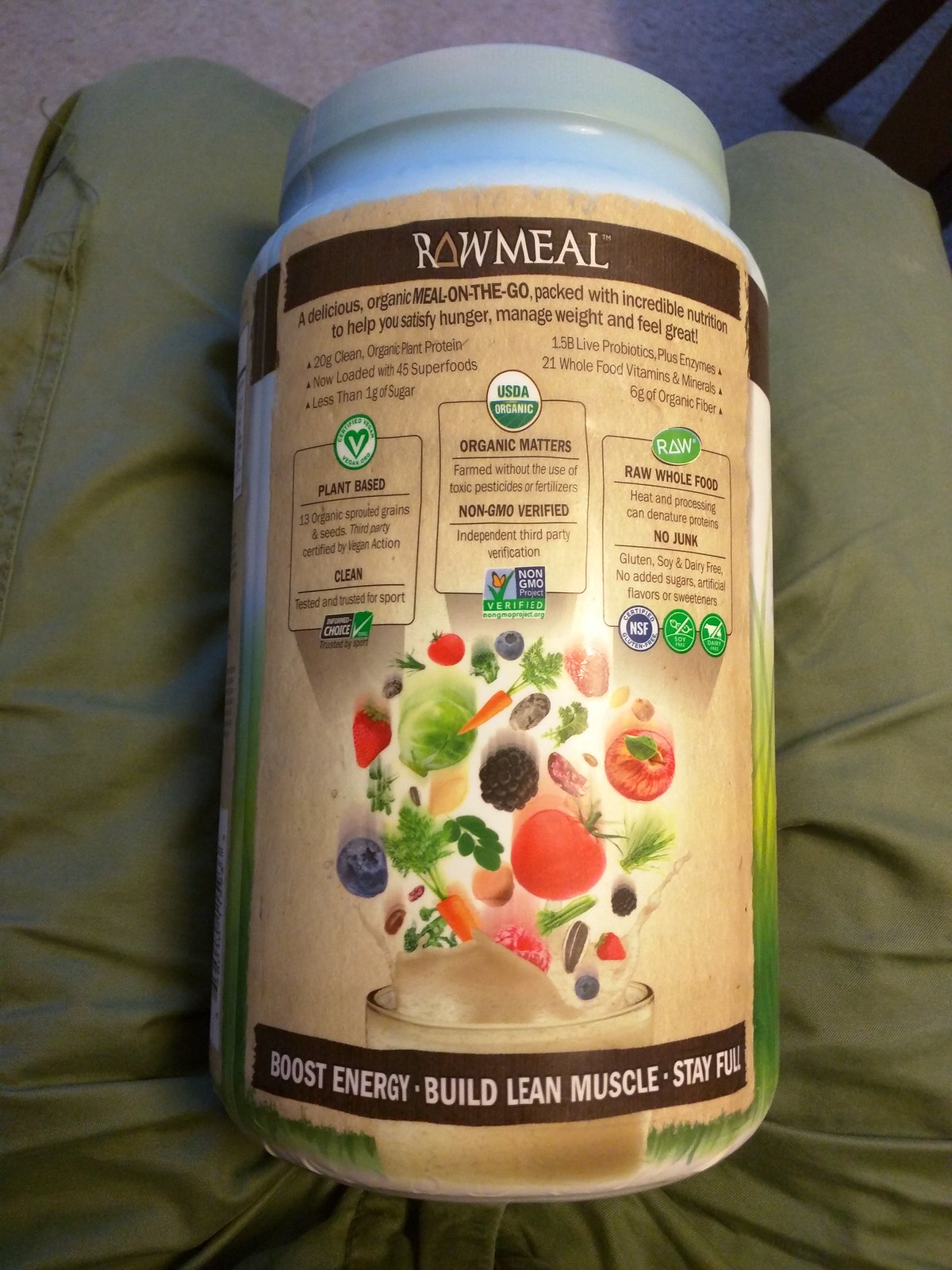The image displays a vibrant arrangement of green plants surrounding a prominently placed jar in the center. The jar features a white lid and a brown label with the words "Raw Meal" written on it. The text on the label reads, "The delicious are going to be on the go. Practically prevalent nutrition," suggesting its convenience as an on-the-go meal solution. Additional text highlights its purpose: "To help you satisfy hunger and manage when you feel grainy."

The jar boasts "45 superfoods," indicating an impressive array of nutrient-dense ingredients. It prominently features the terms "Organic" and "Raw Food," emphasizing its natural and unprocessed nature. A blue circle graphic highlights various fruits and vegetables, including blueberries, a red tomato, and green beans, among others, all dynamically splashing into a rich, brown liquid inside a glass. The product is described as designed to help boost energy and keep you feeling full.